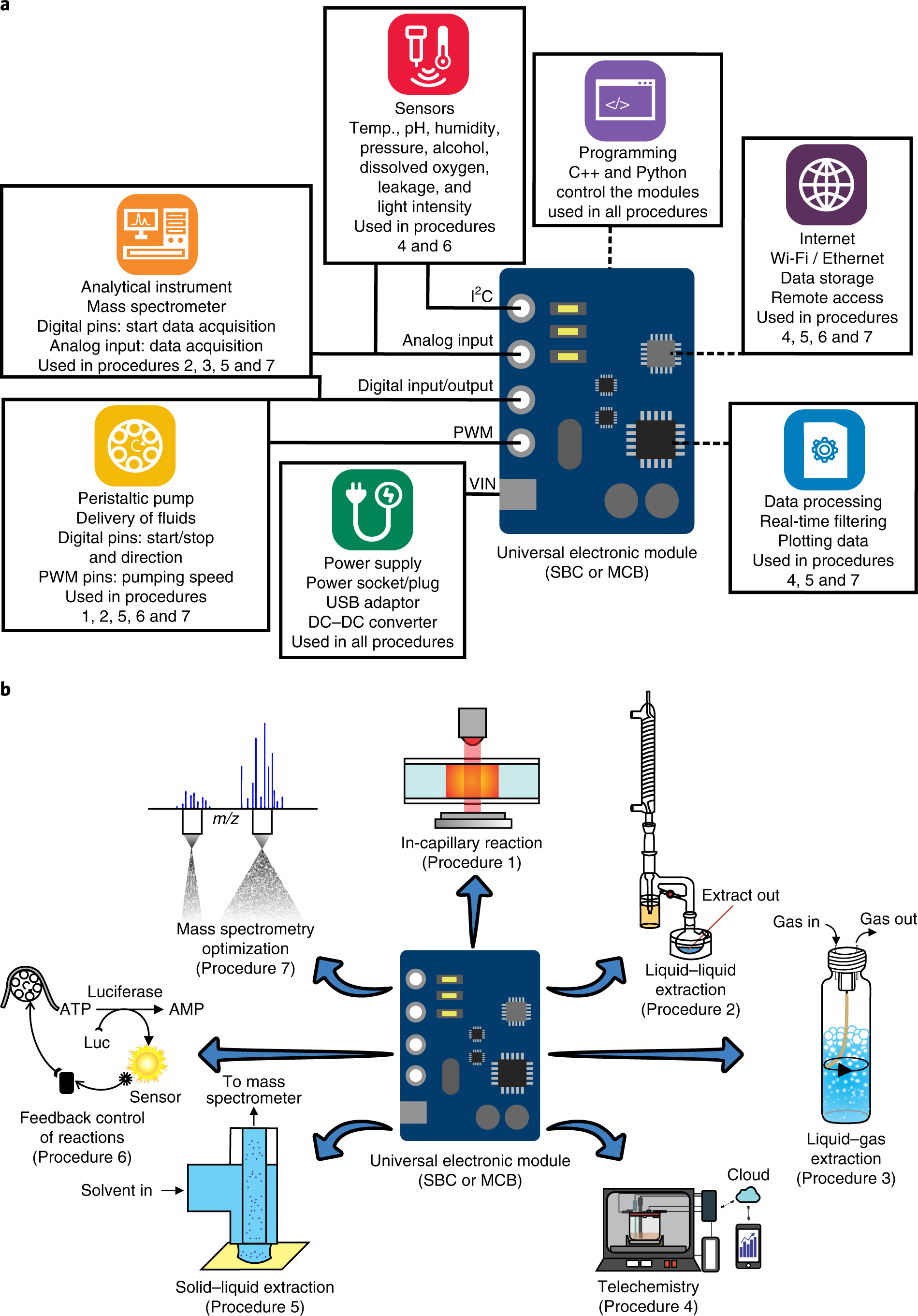This image features detailed flowcharts on a white background, illustrating the functionalities and applications of a Universal Electronic Module (UEM). At the top, a blue circuit board labeled "Universal Electronic Module SBC or MCB" is surrounded by various annotated boxes and graphics. These include:

- A peristaltic pump for fluid delivery, controlled by digital pins for start, stop, and direction, and PWM pins for pumping speed (procedures 1, 2, 5, 6, 7).
- A power plug representing the power supply, including a USB adapter and DC to DC converter, connected above to an analytical instrument mass spectrometer for digital and analog data acquisition (procedures 2, 3, 5, 7).
- Multiple sensors measuring parameters like temperature, pH, humidity, pressure, alcohol, dissolved oxygen, leakage, and light intensity (procedures 4, 6).
- A purple graphic denoting programming capabilities in C++ and Python (use and procedures).
- An icon of a globe indicating internet functionalities like Wi-Fi, Ethernet, data storage, and remote access (procedures 4, 5, 6, 7).
- A chip referencing data processing for real-time filtering and plotting (procedures 4, 5, 7).

The bottom diagram shows the same Universal Electronic Module linked via blue arrows to detailed applications:

- Intercapillary reaction (procedure 1).
- Liquid extraction from a bottle (procedure 2).
- Liquid-gas extraction through a cylinder (procedure 3).
- Telechemistry with cloud integration and smartphone connectivity (procedure 4).
- Solid-liquid extraction (procedure 5).
- A feedback control mechanism involving a LuceraPhase ATP-AMP-LOC sensor (procedure 6).
- Mass spectrometry optimization (procedure 7), displayed with a corresponding chart.

Overall, the image offers a comprehensive exploration of the Universal Electronic Module's circuitry, uses, and procedural applications across various scientific and technological fields.